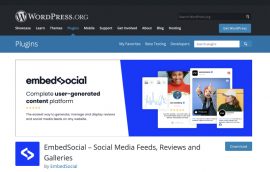A screenshot of a WordPress interface featuring the "Embedded Social" plugin is displayed. The upper part of the screen shows ten navigable sections written in white text. Below this, there is a blue box containing a search bar and three subheadings related to plugins. Within this blue box, there's an image that is half white and half blue, featuring a mix of text and visuals. The text includes black writing and a five-star rating, with descriptions such as "social media feeds," "reviews," and "galleries." The image also depicts various elements, including a child giving a thumbs-up, a mix of people, and some graphical representations. Overall, the screenshot provides a compact but informative overview of what the "Embedded Social" plugin offers.